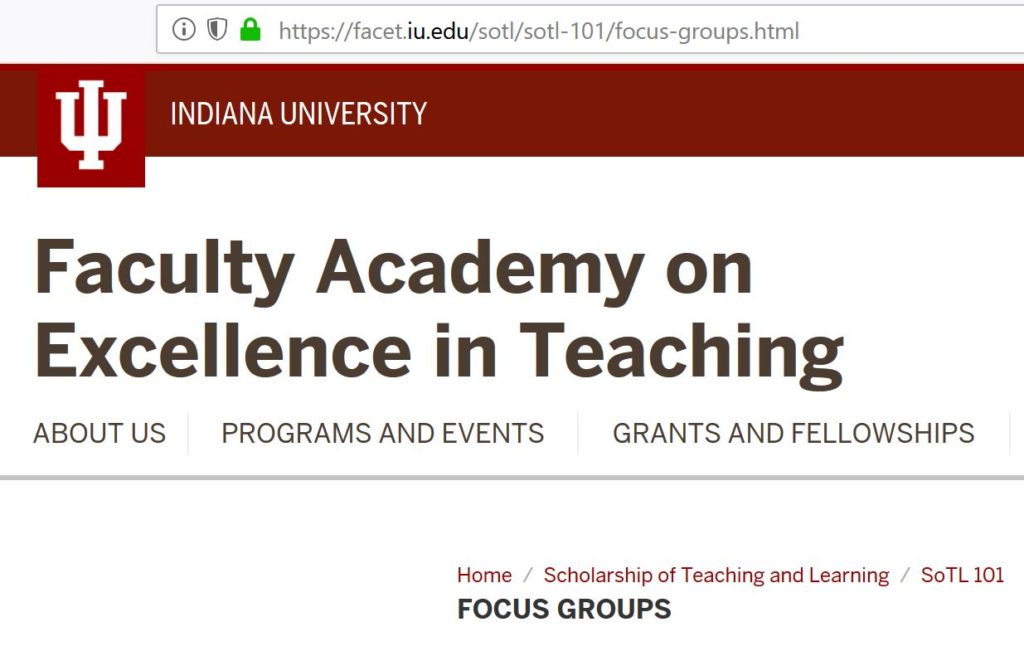The image features a detailed webpage layout:

At the top, a grey background covers the top left portion. Adjacent to it is a white search bar. Next to the search bar, a series of icons appear: a circle with an eye, a shield, and a green padlock. Following the icons is a website address displayed in grey and black text.

Below this, the main section starts with a white background. At the very top, a reddish-brown strip is visible. On the left side of this strip is a unique logo resembling pitchforks; upon closer inspection, it is a stylized overlay of the letters 'I' and 'U', symbolizing Indiana University. To the right of the logo, the words "Indiana University" are written in white text.

On the white background below the strip, "Faculty Academy on Excellence in Teaching" is written in black text. Following this, there is a grey horizontal line. Below the line, a navigation bar in grey text includes the options: "About Us," "Programs and Events," and "Grants and Fellowships."

Towards the bottom right, a breadcrumb trail reads: "Home / Scholarship of Teaching and Learning / TOLT101," where the 'o' is lowercase and the rest are uppercase letters.

Finally, in a bold, dark black font, the text "FOCUS GROUPS" is prominently displayed in all capital letters. The description ends here. 

Moving on to the next section, thank you.